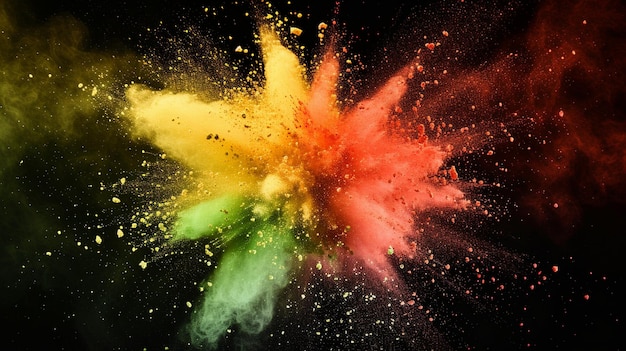The image depicts an otherworldly explosion that resembles a firework composed of colored chalk or smoke against a stark black background. From the center, vibrant streaks and clouds of color radiate outward: the right side showcases hues of red and pink, the upper left erupts in yellow and gold, while the lower left exudes green. This burst generates a smoky, almost cloudy texture, as if chalk dust or fine particles are suspended in the air. Accompanying the main explosion are countless colorful dots and bubbles—red, yellow, and green—scattered in corresponding areas. These minute particles enhance the visual impact, making the colors more striking against the dark backdrop. The entire composition gives off a surreal, perhaps computer-generated feel, capturing the essence of an extraordinary, vividly detailed event in the night sky.